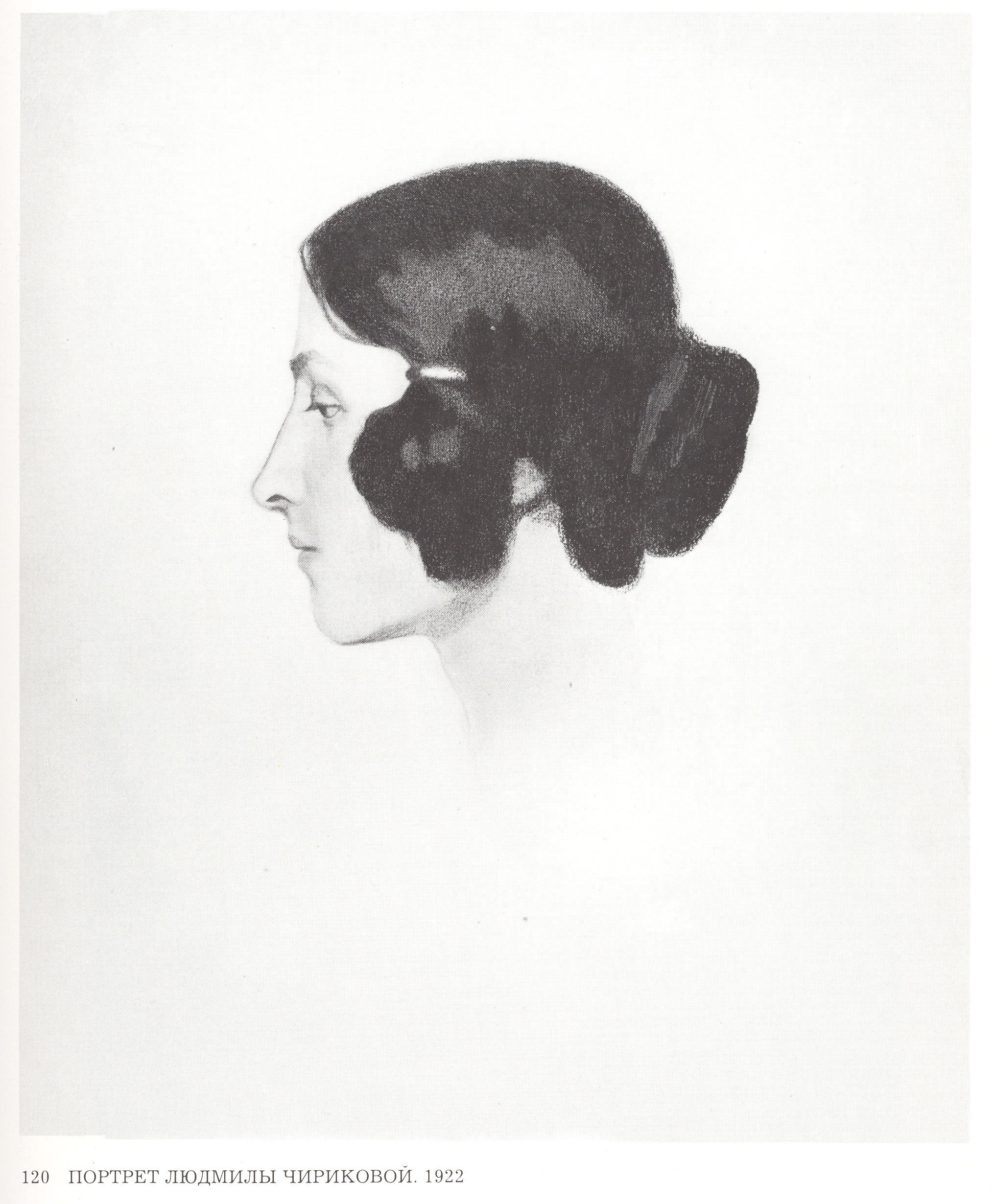This detailed hand-sketched, black-and-white profile portrait from 1922 appears to be an image from a book. The illustration depicts a woman with pale white skin and short, shiny black hair, swept back to the nape of her neck. Her dark hair is gathered at the back, potentially in a bun or a clump, held by a barrette. She has a prominent chin, thin lips, a small angular nose, and a visible single eye with a downward gaze. Her ear is not visible due to the slightly pulled-back hair. In the bottom left-hand corner of the image, the number "120" is inscribed above three words written in what looks like Russian or Cyrillic script, along with the year "1922". The background is a clean white with a lighter white frame around the portrait, adding to its simplicity and focus on the finely detailed features of the woman.